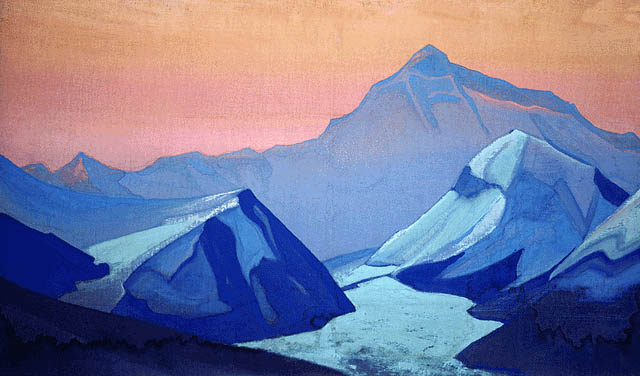This painting captures a mesmerizing natural landscape featuring a series of mountains and a river in the middle, all under a striking sky. The canvas, oriented horizontally, reveals a gradient sky adorned with various shades of reddish pink, peach, and orange, hinting at either sunrise or sunset. Dominating the scene are the sharply defined mountains, layered in different shades of blue. The furthest mountains exhibit a pale icy blue, while those closer range from medium to darker blues, with some peaks accented in turquoise and royal blue. The foreground showcases mountains with hues bordering on navy and royal purple. At the center, a light blue river flows gently between the mountains, appearing almost frozen, suggesting a possible winter scene. Overall, the painting conveys a sense of tranquility through its abstract yet detailed depiction of a serene mountainous landscape.